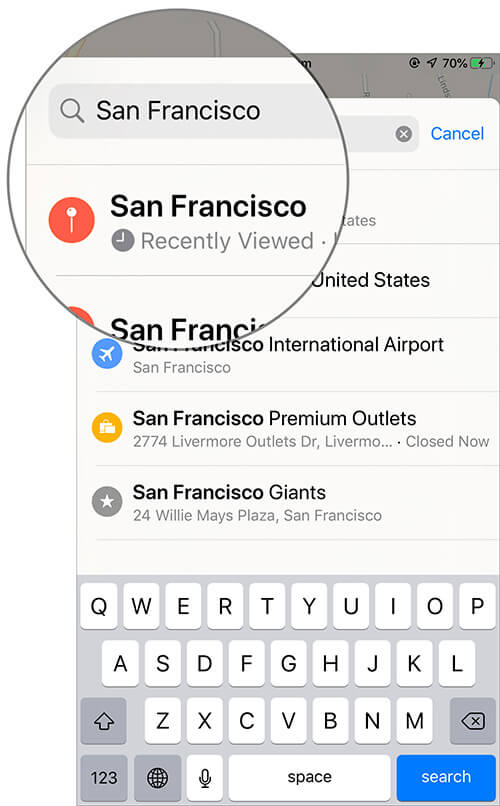This is a screenshot of a mobile phone application interface. The main feature of the image is an enlarged circular magnification in the upper left corner highlighting a specific area of the app.

Inside the magnified circle, the background is light gray. At the top of this section is a medium gray search bar with rounded corners. On the left side of the search bar, there is a dark gray magnifying glass icon, while the right side contains the black text "San Francisco." Below the search bar, there is a thin medium gray line acting as a separator.

Following the separator, there is a search result. This result starts with a pink circle on the left with a white pin icon in its center. To the right of this icon, two lines of text are displayed: the top line is bolded and black, reading "San Francisco," while the line below it is in dark gray and features a clock icon with white hands, along with the words "recently viewed." To the right of this is a small dot. Another thin light gray line beneath this section indicates the edge of the magnified area, where you can see partial text "San France" in bold black and the corner of another pink circle to the left.

The border of the magnifying circle is outlined with a thin dark gray line. Outside the magnified portion, the rest of the app’s interface is visible. The background remains light gray with similar arrangements of search results. To the right of the magnified portion and slightly lower, the text "United States" appears in bold black. Beneath this, another thin gray line separates it from the next entry, which features a blue circle on the left with a white airplane icon, its nose pointing upwards at a 45-degree angle.